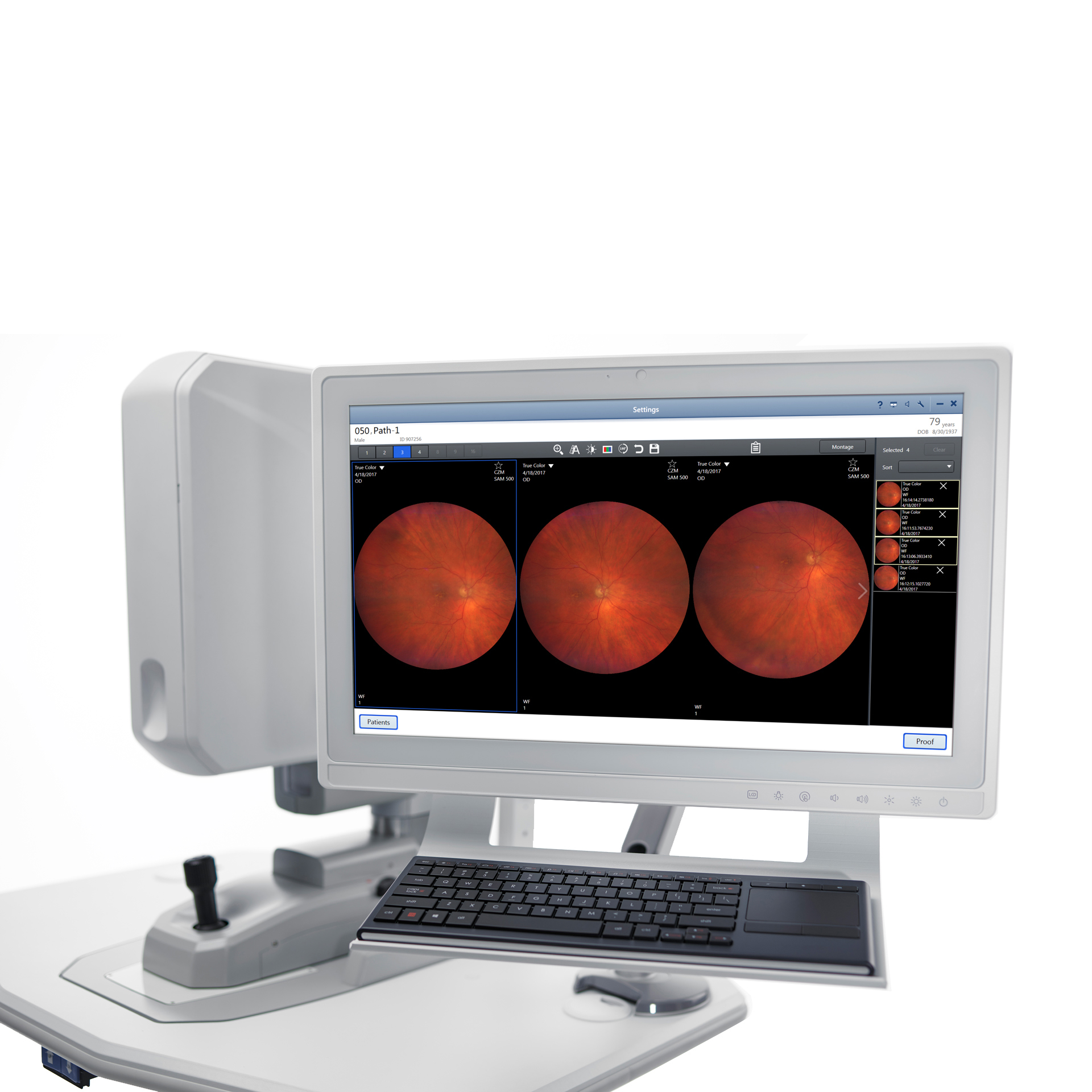This close-up image features a sophisticated medical apparatus, likely an ophthalmic imaging device used to examine and photograph the back of an eye. The device is predominantly white with an attached black keyboard and a joystick to the side, facilitating navigation and interaction with the machine. The monitor, mounted on a white floating table beneath the apparatus, displays various images and detailed slides on a black background, including text such as "OSO 050 Path 1." The red and gray images seem to depict internal structures of the eye, highlighting veins and other features necessary for medical analysis. A divider in front of the monitor prevents patients from viewing the screen directly. The setup is sleek and modern, typical of equipment found in hospitals.